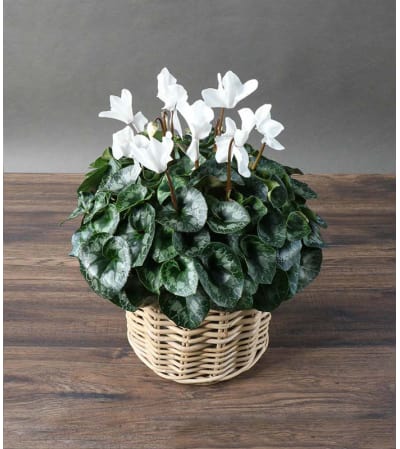The image features a small plant with dark green, variegated, curled foliage arranged in a tightly packed, mounded circular bouquet. Emerging from the lush leaves, there are approximately ten delicate white blossoms, likely of a cyclamen. This arrangement sits in a light beige wicker basket with a coarse weave pattern, placed on a wooden table. The wood has a typical dark brown finish with some darker areas, contributing to the image's vintage quality. The background is a plain gray, ensuring no distractions from the basket and plant. The photograph is focused solely on the basket and its contents, giving it a framed dimension of approximately four inches across by five inches tall. There are suggestions that the plant might be artificial due to its pristine appearance, but the detailed, ornate leaves and flowers contribute to its overall charm.